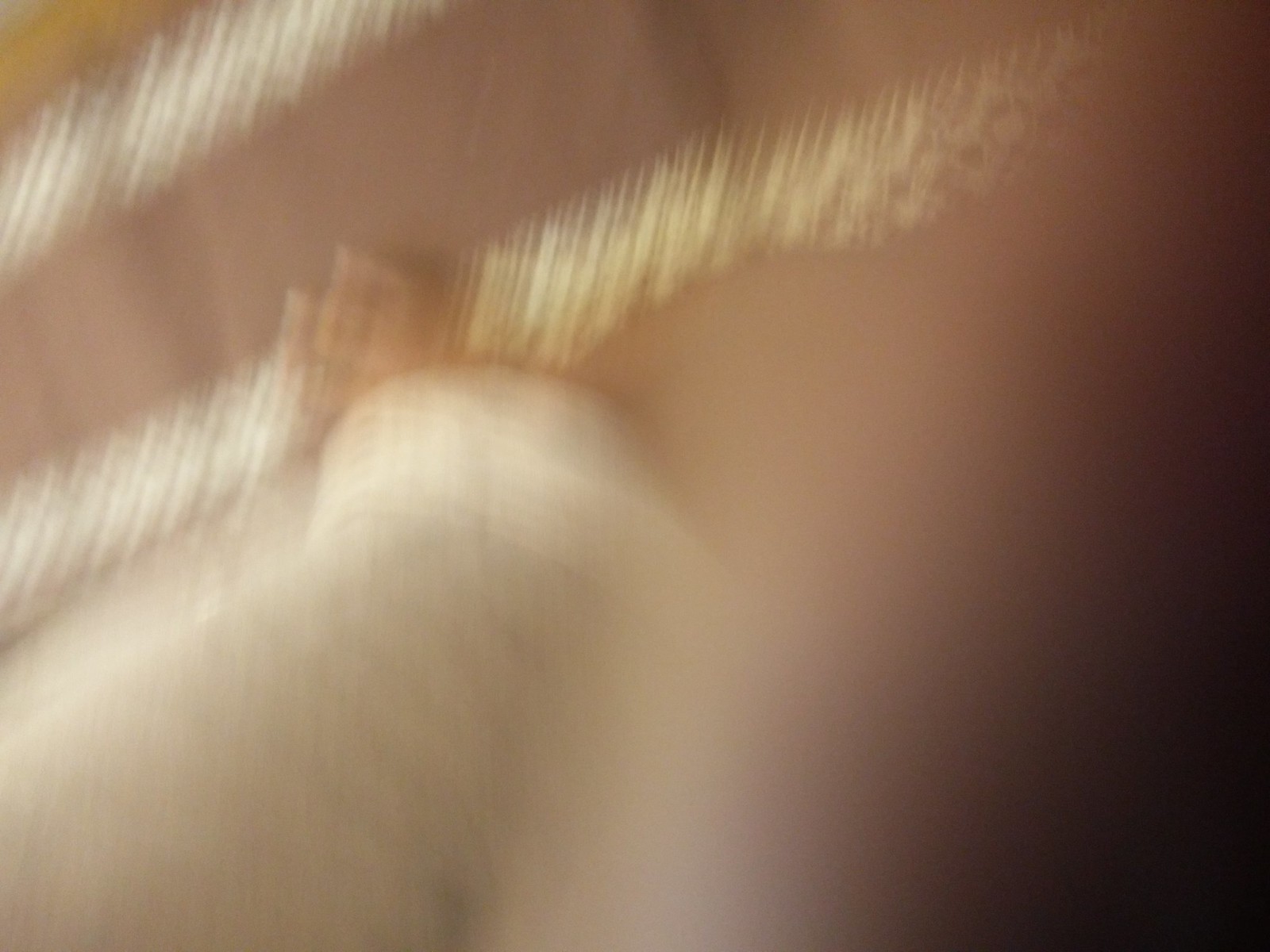The image is an abstract, extremely blurry photograph with predominant beige and tan tones, suggesting it might have been taken accidentally. The central elements include irregular lines and shadows, possibly indicating movement, such as an arm in motion. In the top right corner, there are jagged lines that transition from white to gold, resembling starbursts. The right side features a gradient from black to brown and white. There appear to be some fabric or cloth elements, inserting ambiguity whether it’s a curtain or a t-shirt sleeve. A shadow, potentially someone's finger, extends across the frame, adding to the image's confusing nature. The background might be a sidewalk or tile, implying an outdoor setting with natural afternoon lighting, casting diffuse illuminations throughout.